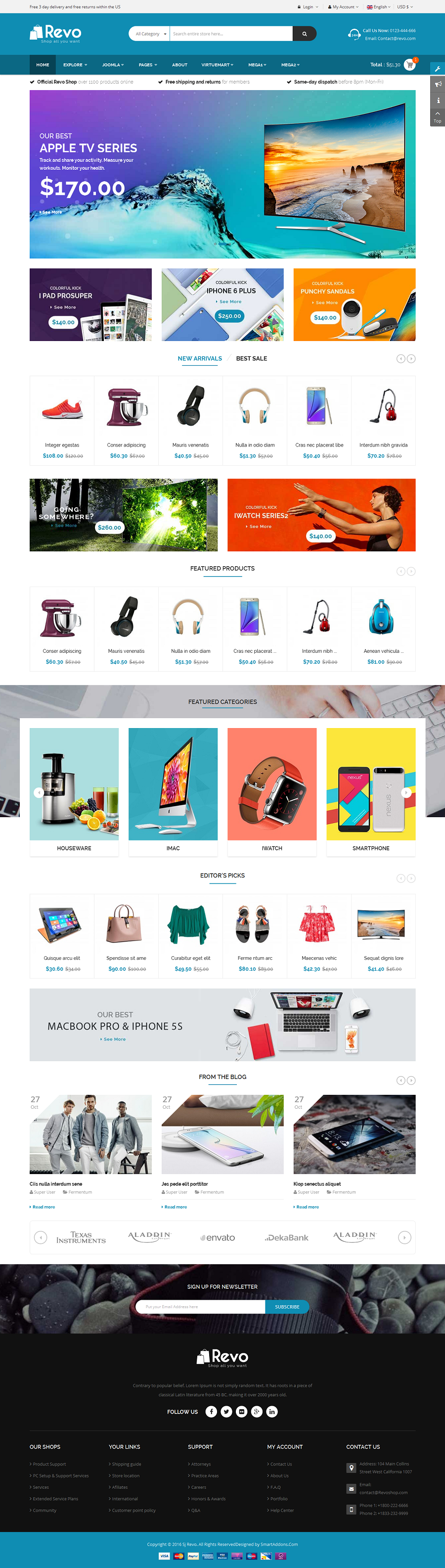This detailed screenshot captures several sections of the Revo website, organized in a vertically scrolling layout. Here’s a comprehensive breakdown starting from the bottom and moving upwards:

1. **Footer Section**: 
   - **Background**: Black
   - **Content**: Displays "REVO" in bold text with navigation links such as Shops, Your Links, Support, My Account, and Contact Us.

2. **Newsletter Signup Section**:
   - **Background**: Image of rocks
   - **Content**: A form inviting users to "Sign up for our newsletter".

3. **Blog Section**:
   - **Background**: White
   - **Content**: Displays images related to blog posts. Notably, the images may not be in English and seem to showcase various purchasable items.

4. **Product Highlight Section**:
   - **Background**: Gray
   - **Content**: Text reading "Our best MacBook Pro and iPhone".

5. **Colorful Product Categories Section**:
   - **Backgrounds**: Includes teal, dark teal, orange, and yellow
   - **Content**: Features products like houseware, iMac, iWatch, and smartphones.

6. **Featured Categories Section**:
   - **Content**: A bordered heading "Featured Categories".

7. **Featured Products Section**:
   - **Content**: Highlights various featured products with accompanying images.

8. **Scenic Image Section**:
   - **Content**: Displays both an outdoor scene and an indoor scene, followed by more product images categorized as "new arrivals" and "best sale".

9. **Promotional Products Section for Apple Products & Accessories**:
   - **Content**: Includes detailed promotional content and images for products like iPad Pro, iPhone 6 Plus, and Punchy Sandals.

10. **Apple TV Series Promotion**:
    - **Content**: Boasts a "Great big TV for $170", speculated to possibly be a monitor.

11. **Website Identification**:
    - **Position**: Upper left-hand corner
    - **Content**: Indicates the website being viewed is the Revo website.

These clearly segmented sections build a comprehensive and detailed representation of the Revo website screenshot.